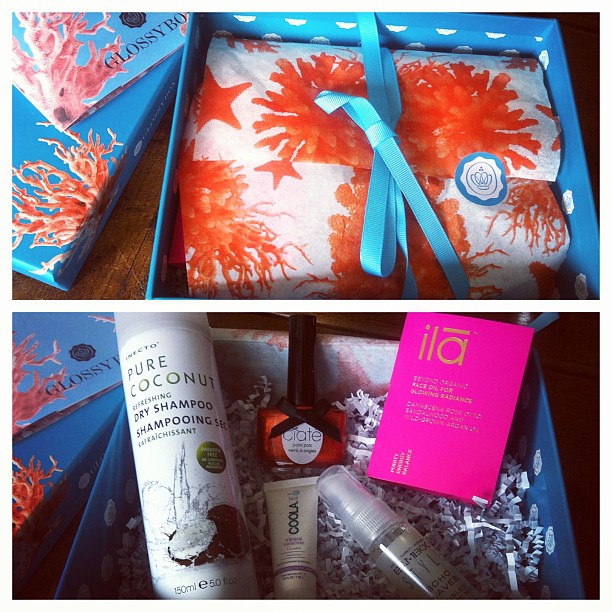The image is a square composed of two evenly divided photographs, separated by a white line. The top photograph features an open blue box adorned with ocean scenery on the outside. Inside the box, a glossy book and a white towel with ocean-themed designs in orange are neatly nestled. The towel is secured with a blue ribbon and there are two red and white wrapped items inside as well.

In the bottom photograph, we see the same blue box without the wrappings. The contents are clearly displayed: a bottle of Pure Coconut Refreshing Dry Shampoo with an illustrative coconut image, a tube of cocoa hair gel, a spray, a perfume bottle, and a soap labeled "Ciate," which is red with a black ribbon against a white background. The box rests atop another box filled with shredded paper, adding a touch of texture to the presentation. This collection of health and beauty products is carefully arranged in a visually appealing manner.